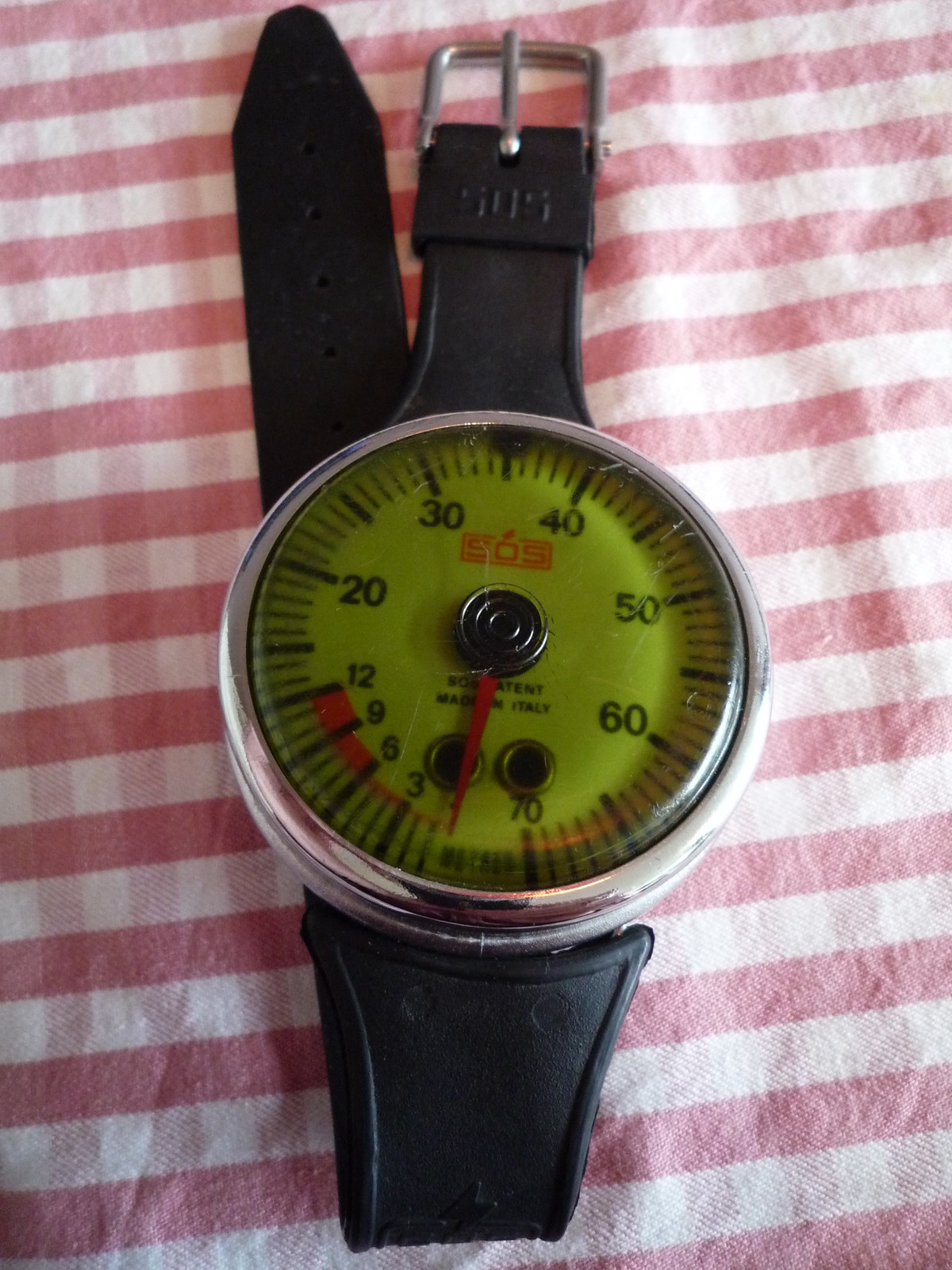This close-up photograph captures a unique wrist-mounted device positioned against a vibrant checkered tablecloth featuring red, white, and light red plaid patterns. The device sports a black silicone band with a silver buckle, folded in half with its face prominently displayed. Encased in a sleek silver housing, the face of the device showcases a distinctive pea green background with black markings ranging from 0 to 70. At the top of the display, a red box encloses the bold letters "SOS" in red. A single red needle dominates the center of the face, pointing precisely at a marking. Beneath the needle, the words "SOS patent" and "made in Italy" are visible, further indicating this is not an ordinary wristwatch but rather a specialized piece of equipment designed for specific purposes.